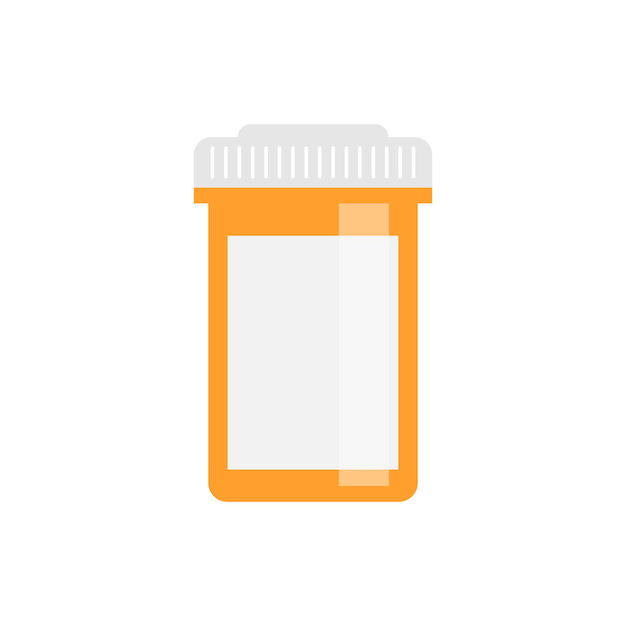The image depicts a digitally created or hand-drawn representation of a rectangular-shaped medicine pill bottle. The bottle, which lacks any written label or text, showcases a blank, white rectangular label on its front, creating a see-through section amidst the predominantly orange body. The orange color appears darker at the bottom and gradually lightens towards the top where a lid is present. The white or light gray lid features around 15 thin slots or ridges, resembling air vents. The overall design of the bottle is rendered in a side view, standing upright, emphasizing realistic proportions and detail.